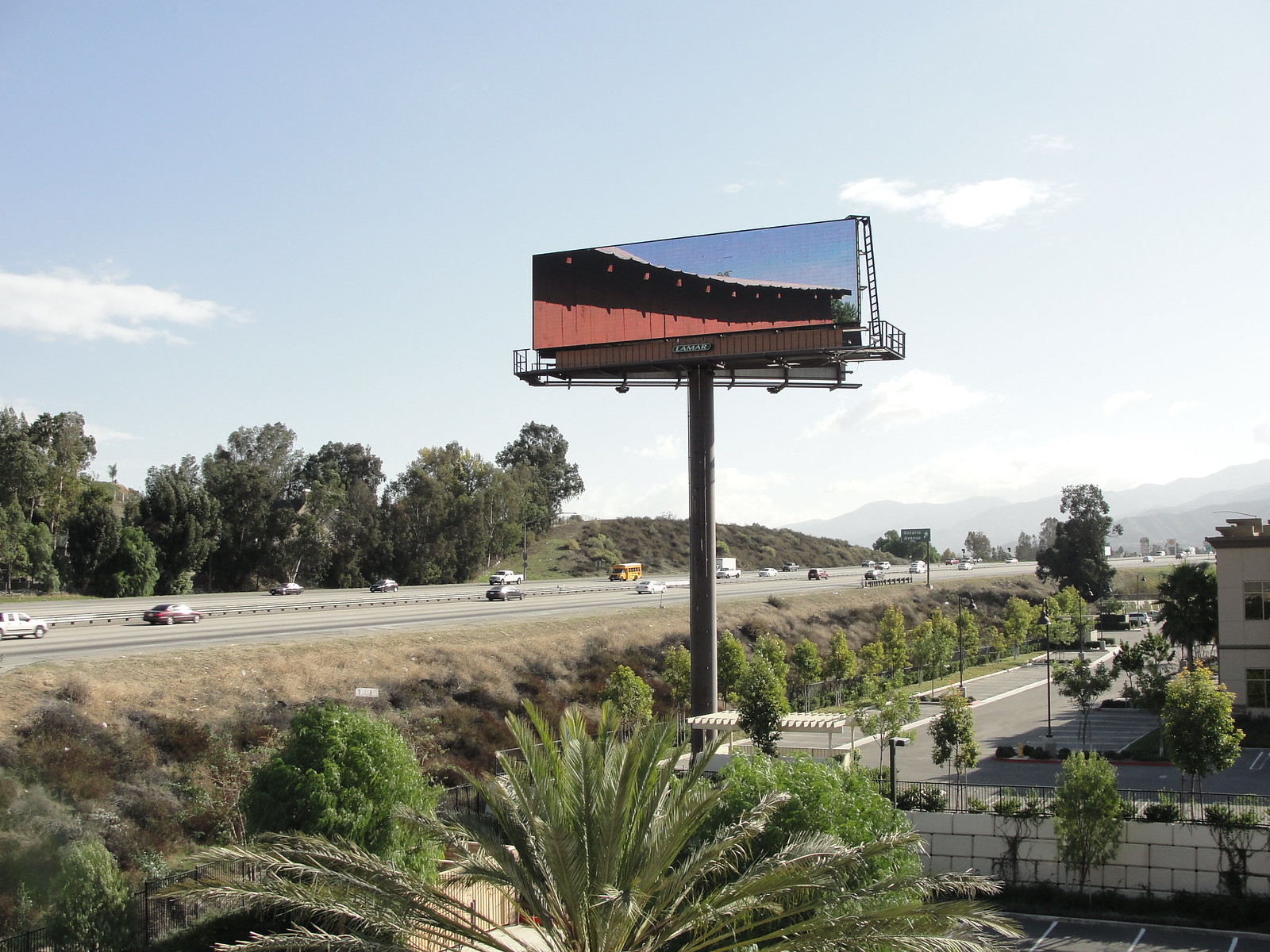A vivid freeway scene features a prominent billboard positioned centrally between a bustling freeway to the left and a smaller road to the right. The billboard showcases a swirling pattern of red, pink, and blue lines that gracefully spiral from the top left to the bottom right. In the foreground, a grove of tall, lush palm trees lines the side of the road, adding a touch of greenery to the scene. The freeway is crowded with approximately 20 vehicles, suggesting a high traffic volume. In the distance, the rooftops of residential houses peek out, hinting at a nearby neighborhood. The sky above is a clear, bright blue with just a few wispy clouds, and the sunlight, coming from the right of the image, bathes the entire scene in a warm, natural glow.